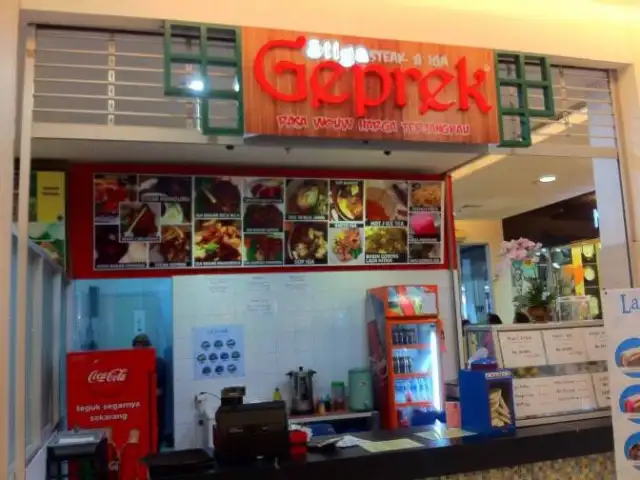The image showcases a vibrant food kiosk storefront. The signage features a distinct brown wooden board framed in green with stylized red lettering that reads "Geprek," and above it, illuminated text says "Stiga Steak". The sign is complemented by additional, less legible verbiage. Below this prominent signage hangs a large menu board divided into several panels, each depicting assorted food items with descriptions. The counter area beneath the menu is black and houses a black cash register along with a blue dispenser and some paper on a glass window. The left side of the kiosk features a red Coca-Cola cooler, while behind the counter, there's another red beverage cooler with multiple shelves filled with beverages next to a green beverage dispenser and a metal and black coffee pot. The overall setup suggests a bustling spot designed to attract customers with its colorful and detailed display.